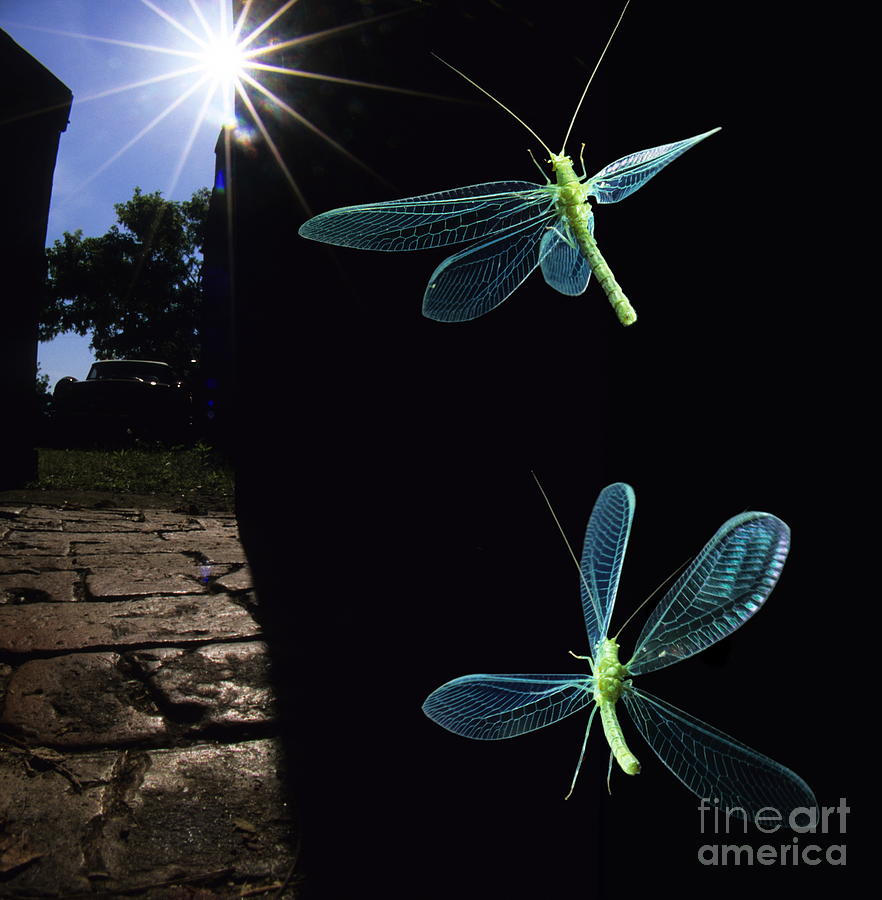The image is a square-shaped, realistic photograph that appears to be taken outdoors, possibly intended as an advertisement for Fine Art America, indicated by the faded white script in the bottom right corner. The composition is split dramatically with a sunlit scene on the left and a nearly pitch-black backdrop on the right. On the left, we see a brightly lit garden featuring a blue sky, a sunburst, and shadows cast by the sun behind, and a tree with a shadowed canopy. On the ground, there is a red-bricked walkway or patio and possibly a car parked on some grass. On the contrasting dark right side, which might be a shadow or digitally edited black background, two vividly colored, dragonfly-like insects with green bodies, blue wings, and green antennas are in flight. The insects, appearing almost computer-animated, seem to be flying towards the viewer, adding a touch of surrealism to the natural setting.